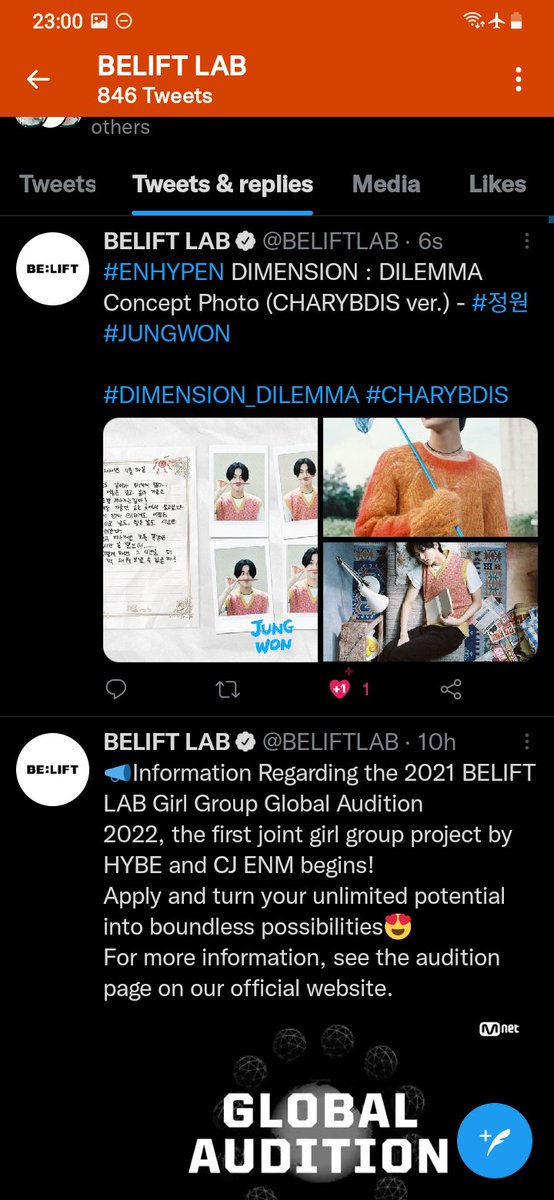In this screenshot of a cell phone display, we see two tweets from a company named Beelift Lab. The top of the screen features an orange header. On the top left corner, the current time is displayed as 23:00. On the right side of the header, a Wi-Fi icon and a battery indicator, showing half charge, are visible.

Beneath the header is the Beelift Lab profile section, containing a white circle with "Beelift" written in the center, followed by the text "Beelift Lab, 846 tweets." Below this, there are four selectable categories: Tweets, Tweets & Replies, Media, and Likes. The "Tweets & Replies" category is highlighted in white with a blue line underneath, indicating it is currently selected.

The first tweet at the top displays the Beelift Lab profile picture and mentions that the tweet was posted six seconds ago. The tweet reads: 
"#-dimension dilemma concept photo" and refers to two attached photos. It includes three hashtags: #dimension, #dilemma, and #cherrybuds (not cherry biddes). It has received one like. The tweet elaborates:
"Information regarding the 2021 Beelift Lab girl group global audition 2022. The first joint girl group project by Hive and CJ ENM begins. Apply and turn your unlimited potential into boundless possibilities. 👁️ For more information, see the audition page on our official website."

At the bottom of the screen is the text "global audition" alongside a blue circle icon to add a new tweet.